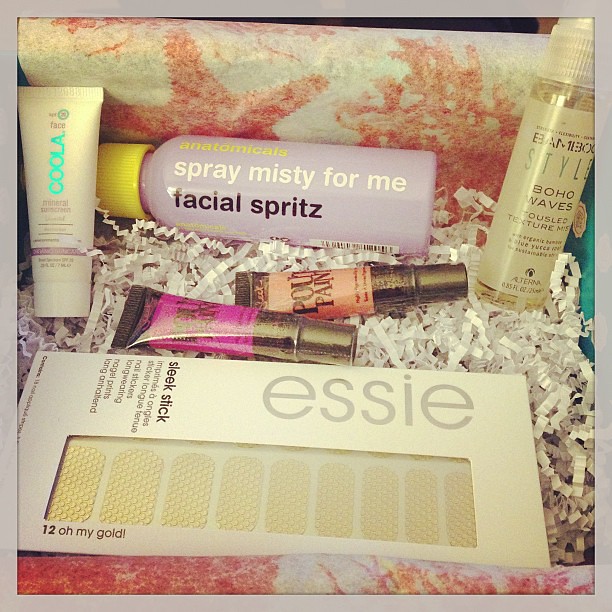This image showcases the contents of an open gift box filled with beauty and self-care products, nestled in a bed of shredded, crinkled white paper. In the upper left corner, there is a white bottle labeled "Face Coola Mineral Sunscreen." Next to it, in the very back, stands a pink and purple bottle with a yellow cap that reads "Spray Misty For Me Facial Spritz" by Anatomicals. To the right of that is a yellow bottle with a clear cap labeled "Bamboo Style Boho Waves Tousled Texture Mist" by Alterna. In the mid-ground, there are two smaller bottles; one has a peach hue with a gold cap, and the other is pink with a gold cap, though their contents are not specified. Positioned centrally are two small clear tubes with black caps, each labeled "Pout Paint"—one containing a purple product and the other a peachy-brown one. Finally, in the foreground, there is a sleek white box with a clear window showing nail stickers adorned with small gold dots from the Essie brand, labeled "Sleek Stick, 12 Oh My Gold." The background of the box features light-colored tissue paper with peachy coral sea life designs, including a sea star and a piece of coral.